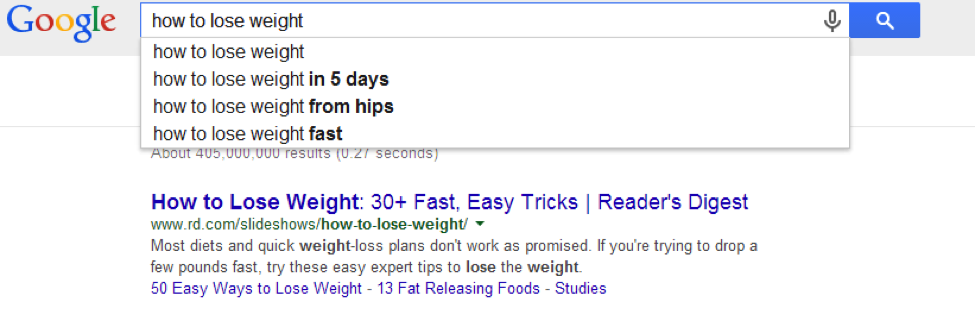A landscape-mode screenshot featuring a Google search page. At the upper left, the familiar Google logo is displayed prominently next to an active search bar, where the user has typed "how to lose weight." Below the search bar, Google suggests related queries: "how to lose weight," "how to lose weight in five days," "how to lose weight from hips," and "how to lose weight fast." 

To the upper right of the search bar, there is a blue magnifying glass icon to initiate the search and a microphone icon for voice searches. The search results indicate approximately 450 million results retrieved in 0.27 seconds.

The top search result, which the user has yet to click, is highlighted in blue and reads "How to Lose Weight: 30+ Fast, Easy Tricks," from Reader's Digest. The URL beneath it is rd.com/slideshow/how-to-lose-weight, suggesting the content is presented in a slideshow format. The snippet offers a brief overview: "Most diets and quick weight loss plans don't work as promised. If you're trying to drop a few pounds fast, try these easy expert tips to lose the weight."

Below this snippet, three related links are shown: "50 Easy Ways to Lose Weight," "13 Fat-Releasing Foods," and "Studies." The detailed view exemplifies a typical Google search results page for weight loss tips, providing a comprehensive set of options for the user to explore.